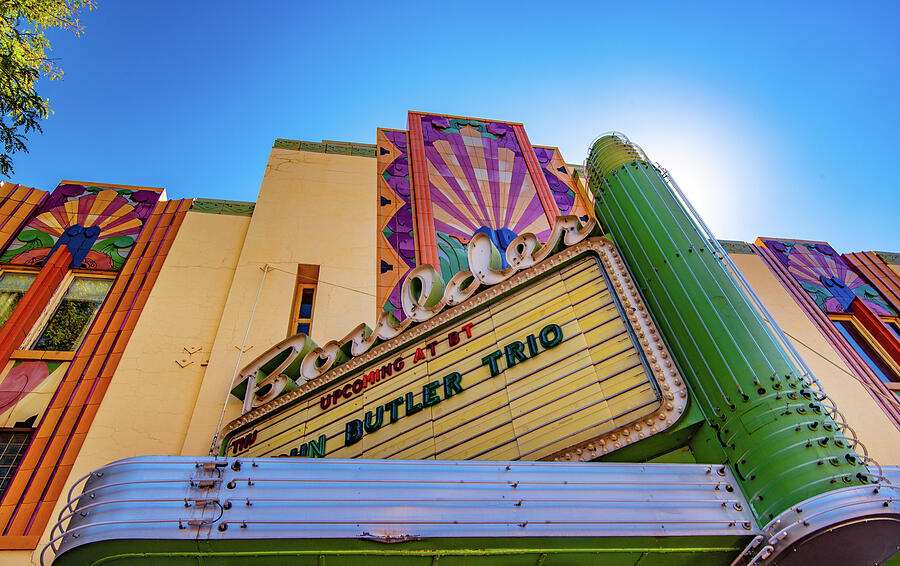The photograph features a vibrant, vintage art deco movie theater named "Boulder," captured from a ground-up perspective against a clear, bright blue sky. The theater's marquee, painted yellow, displays the text "Upcoming at BT" with the notable mention of "John Butler Trio." The theater’s facade is adorned with bright colors, including a predominant yellow and green exterior, complemented by accents of purple and orange. Above the marquee, a yellow starburst adds a dynamic flair, while a giant green cylindrical light fixture with a yellow top stands prominently to the left. Below the marquee, a horizontal metal strip lends to the retro aesthetic. The building's architecture is further emphasized by neon lights running both horizontally and vertically, likely illuminating the theater strikingly at night.